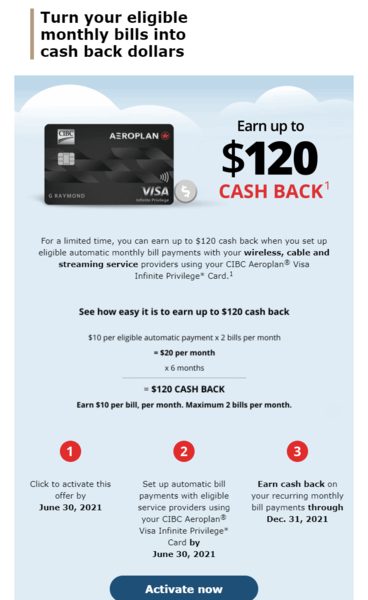**Image Caption:**

The image showcases an advertisement, likely displayed on a mobile device, aimed at promoting a financial offer. The top of the advertisement features the text in bold black, "Turn your eligible monthly bills into cash back dollars." Below this text, a Visa credit card is prominently displayed, branded with both the Aeroplan logo in the top right corner and the CIBC logo in the top left.

Adjacent to the Visa card, on the left, there's a gray circle icon with a white dollar symbol inside. Next to this icon, the text reads, "Earn up to $120 cash back," alongside a small number "1," indicating that terms and conditions apply.

Below this, the advertisement provides further details: "For a limited time, you can earn up to $120 cash back when you set up eligible automatic monthly bill payments with your wireless, cable, and streaming service providers using your CIBC Aeroplan Visa Infinite Privilege card."

Further down, the ad mentions "other ways to earn money" and provides instructions on how to set up the card. At the bottom of the image, a prominent blue button with the text "Activate" encourages users to take action and activate their card.